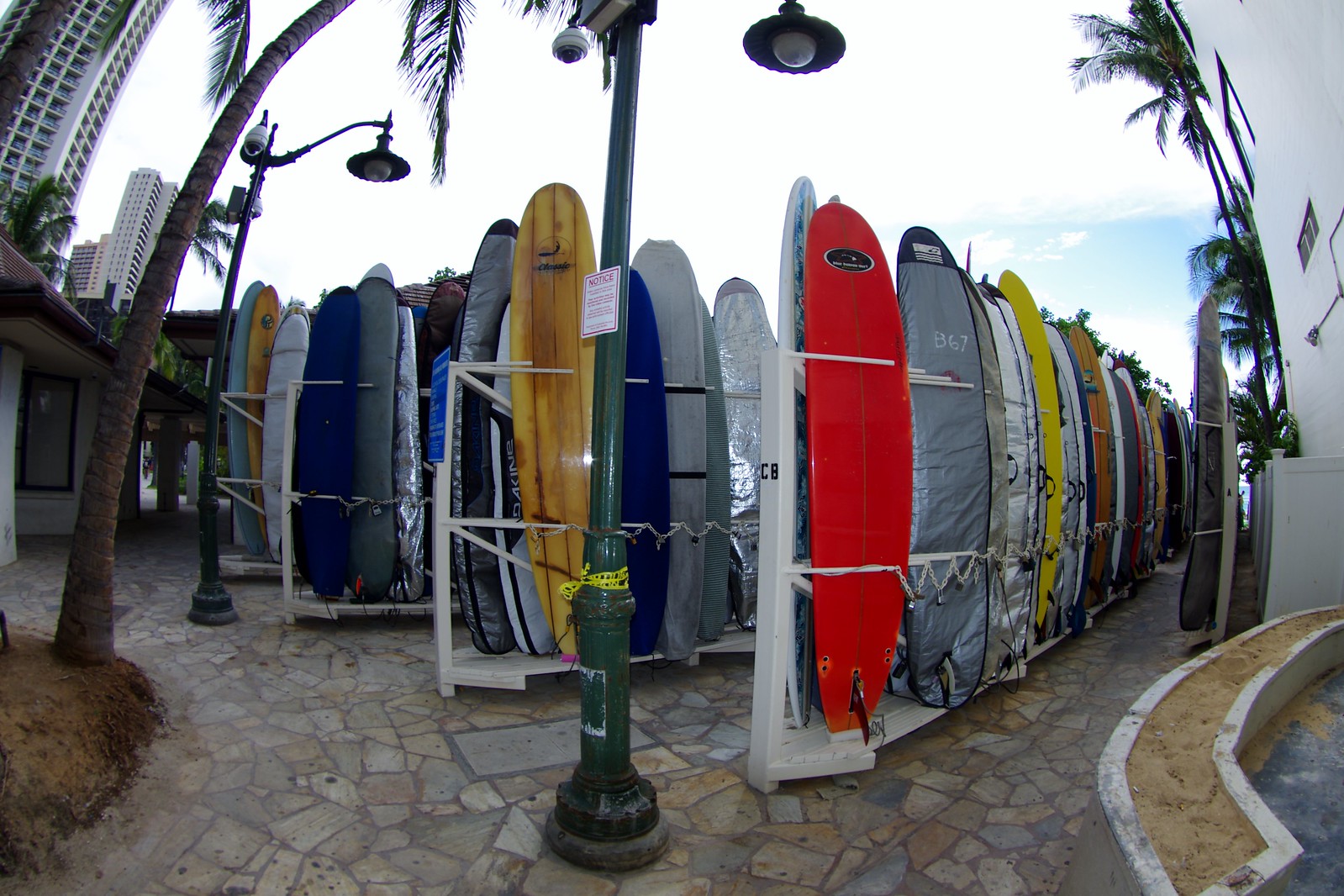This detailed outdoor photograph captures a vibrant array of surfboards meticulously lined up in four rows, held upright by white racks. The surfboards, which number over 25, exhibit a spectrum of colors including blue, yellow, red, grey, green, black, and plain designs. The bright red surfboard stands out prominently. They rest on a surface of cobblestone-like paving stones, crisscrossed with dark grout. 

Dominating the center is a sturdy green metal light post, adorned with a yellow piece of tape or ribbon tied into a bow and a small white sign with unreadable writing. The pole is equipped with a lantern-style light and additional elements that could include a camera.

In the background, a blue sky with scattered white clouds extends above the scene, with a white wall marking the right edge. Tall buildings, possibly hotels with numerous windows, occupy the upper left corner, their heights partly obscured by the frame. A distinctive wide-angle lens effect slightly curves the edges of the image.

Vegetation enhances the outdoor setting: a palm tree on the left side arcs its leafy fronds over some surfboards, while another tree appears in the distant right background. Overall, the image harmoniously blends elements of urban architecture, natural scenery, and the colorful surf culture, framed by a sky transitioning between clear blue and cloud-filled white.